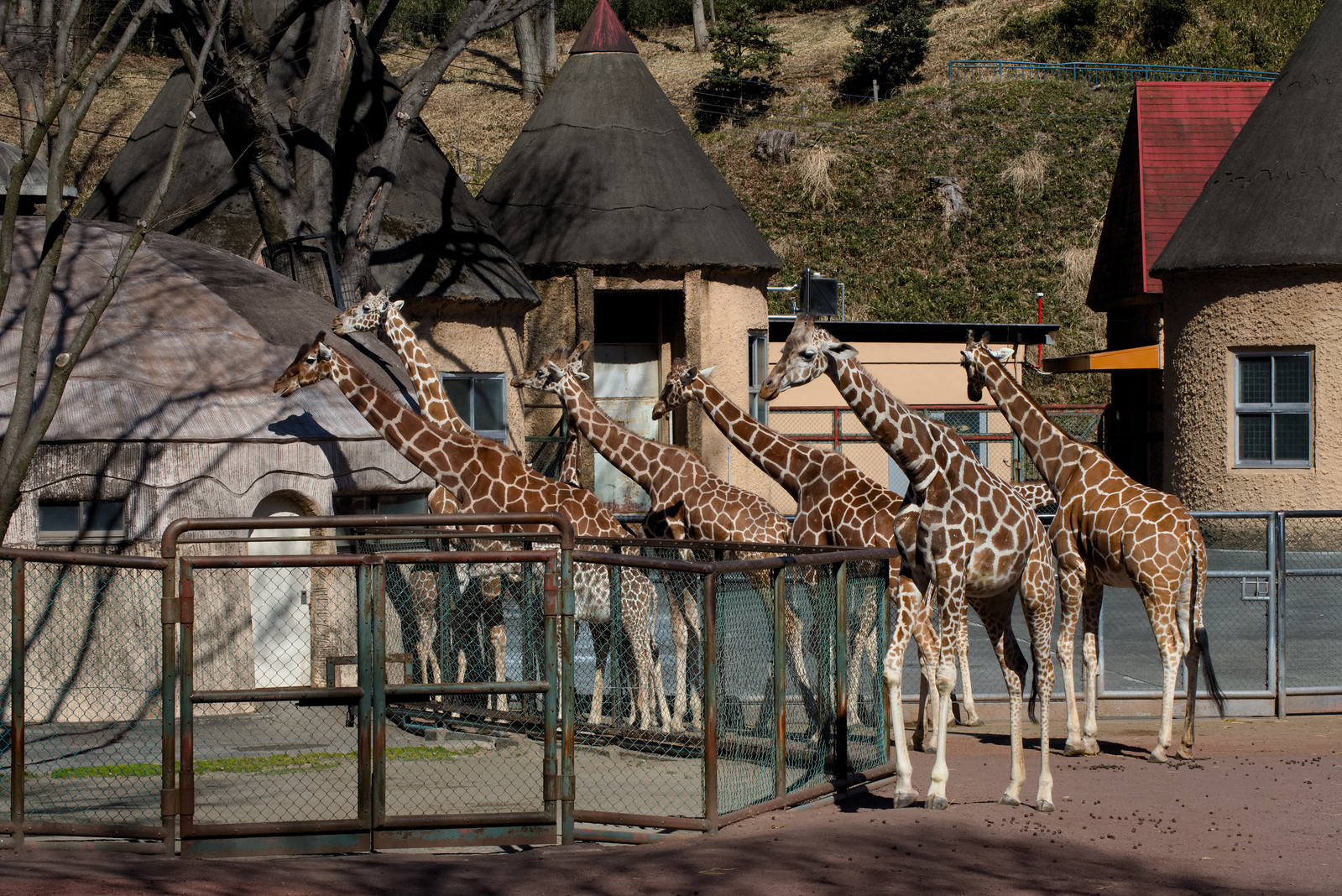In the fenced-in zoo enclosure with a rusty gate, six giraffes of varying shades of brown stand together, all facing to the left. While most of the giraffes are a consistent brown color, one on the right is notably darker. The ground is dirt, and to the left, there's a barren tree in the foreground. In the background, a series of buildings are visible: one with a light gray structure and dark gray roof, another with a red roof, a cream-colored building with a gray roof, and a completely light gray building. The very back of the scene features a large grassy hill dotted with green bushes and trees. No other animals are present in the frame, and the giraffes vary slightly in size, though none appear to be babies.